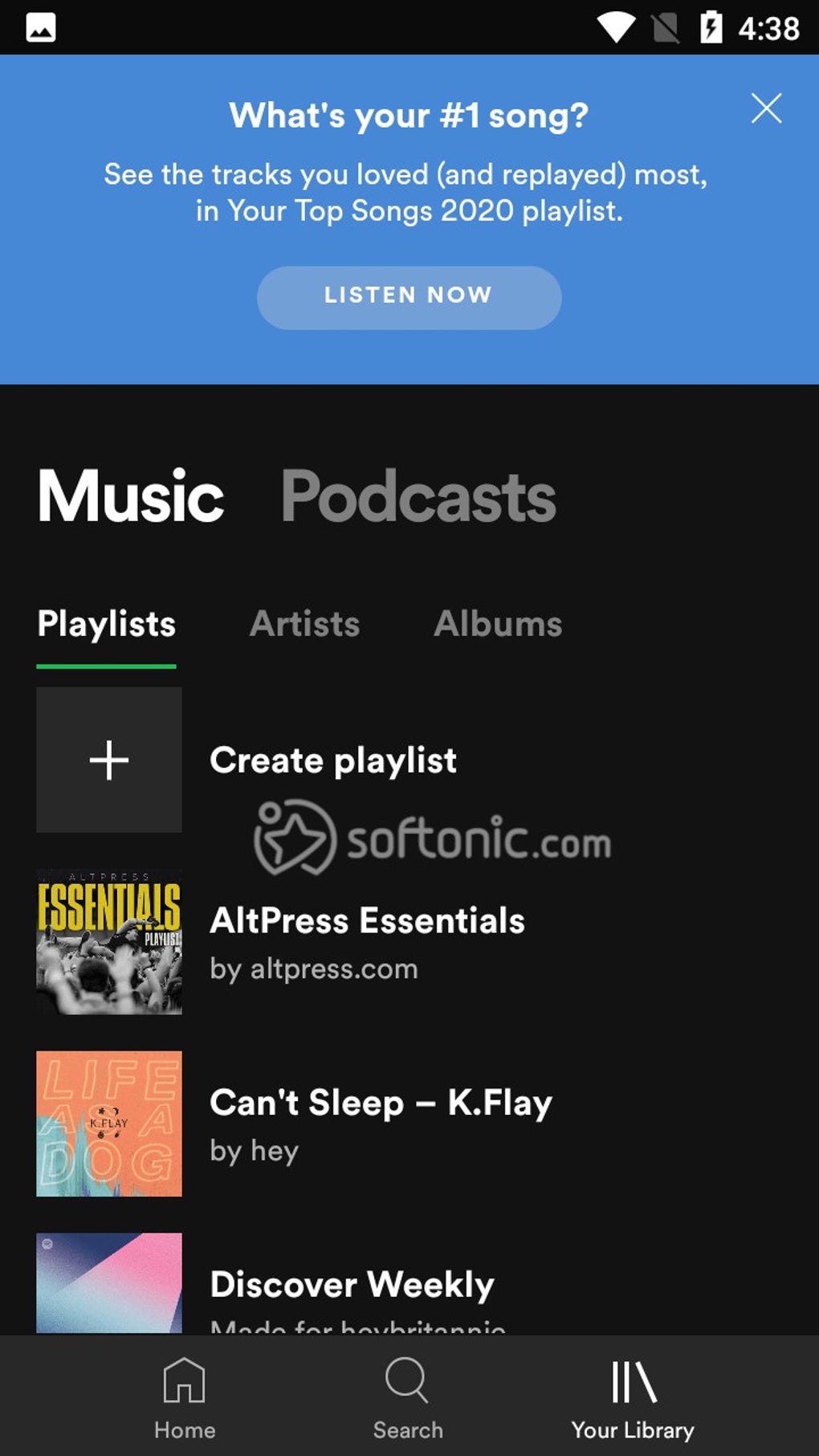This vertical screenshot was captured on a mobile device, showcasing a Spotify interface. The device has a fully charged battery currently being charged and the time indicated is 4:38. Prominently displayed at the top of the screen is a blue notification box with white text, asking, "What's your number one song? See the tracks you’ve loved and replayed most in your Top Songs 2020 playlist." To the right of this message is a small 'X' icon for closing the notification. At the bottom of the blue box, a light blue button with the words "LISTEN NOW" in all capital letters invites user interaction.

Below this notification appears part of the Spotify app's user interface, characterized by a black background. On the left, "Music" is highlighted in large white letters, while "Podcasts" appears in gray to the right. Underneath, the white text "Playlists" is underlined in green, signifying it as the currently selected tab. Adjacent tabs, "Artists" and "Albums," are displayed in gray and positioned to the right.

Navigating further down, there is a gray box with a plus sign and the text "Create Playlist," suggesting an option to create a new playlist. Notably, a faint watermark reading "softtonic.com" with a star surrounded by a circular line appears alongside this box.

Below the watermark, the interface lists playlists with associated creators and titles: "AltPress Essentials" by altpress.com, "Can't Sleep, K.play" by Hey, and "Discover Weekly." At the very bottom of the screen, the navigation bar includes icons for "Home," "Search," and "Your Library," essential tools for navigating the Spotify app.